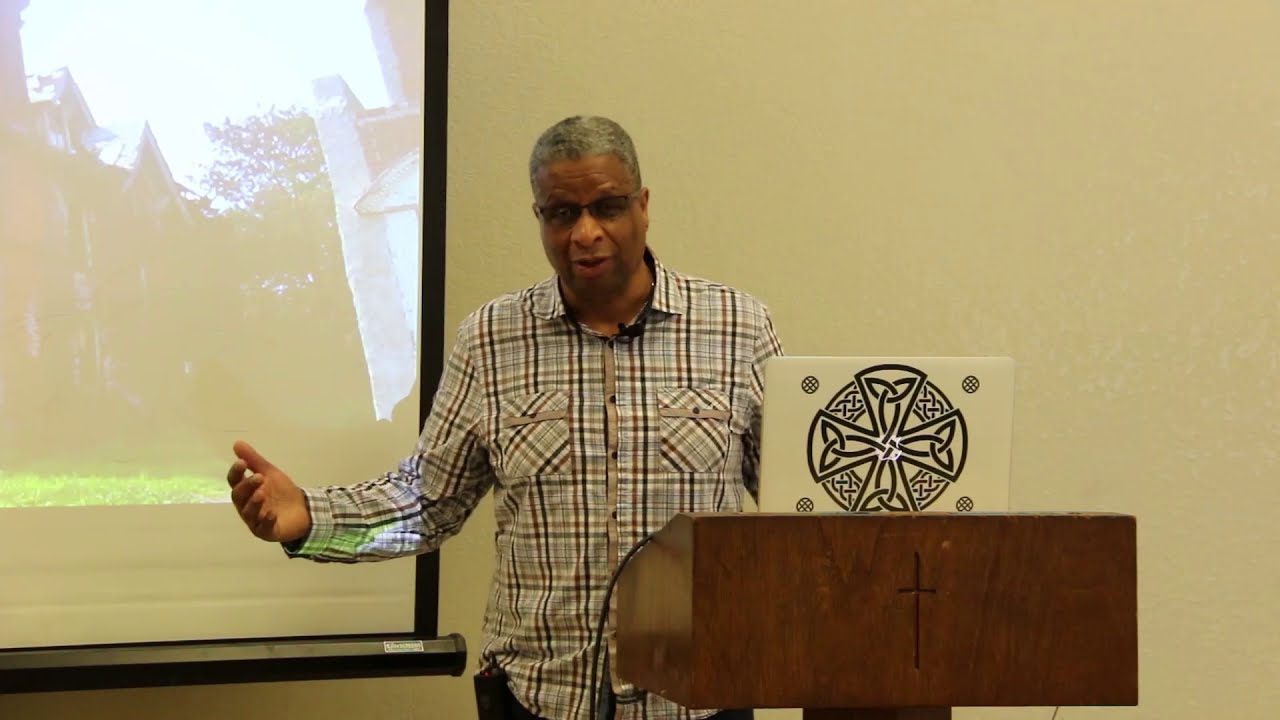The image depicts an older African American gentleman standing behind a wooden podium with a cross etched into the front, suggesting the setting might be a church or a classroom. The man, wearing black-rimmed glasses, a small clip-on microphone, and a long-sleeved plaid shirt in shades of brown, blue, and tan, has short cropped, salt-and-pepper hair. He is extending his right arm outward as he addresses an unseen audience.

Atop the podium is a laptop with a circular decal resembling a Celtic-style cross. There are wires hanging from the podium, likely for the microphone or laptop. The background features an off-white, yellowish wall and a projection screen to the man's right, displaying a slightly washed-out image of buildings, trees, and yards, possibly a neighborhood scene.

The detailed setting highlights a serene indoor environment, potentially during a presentation or lecture.